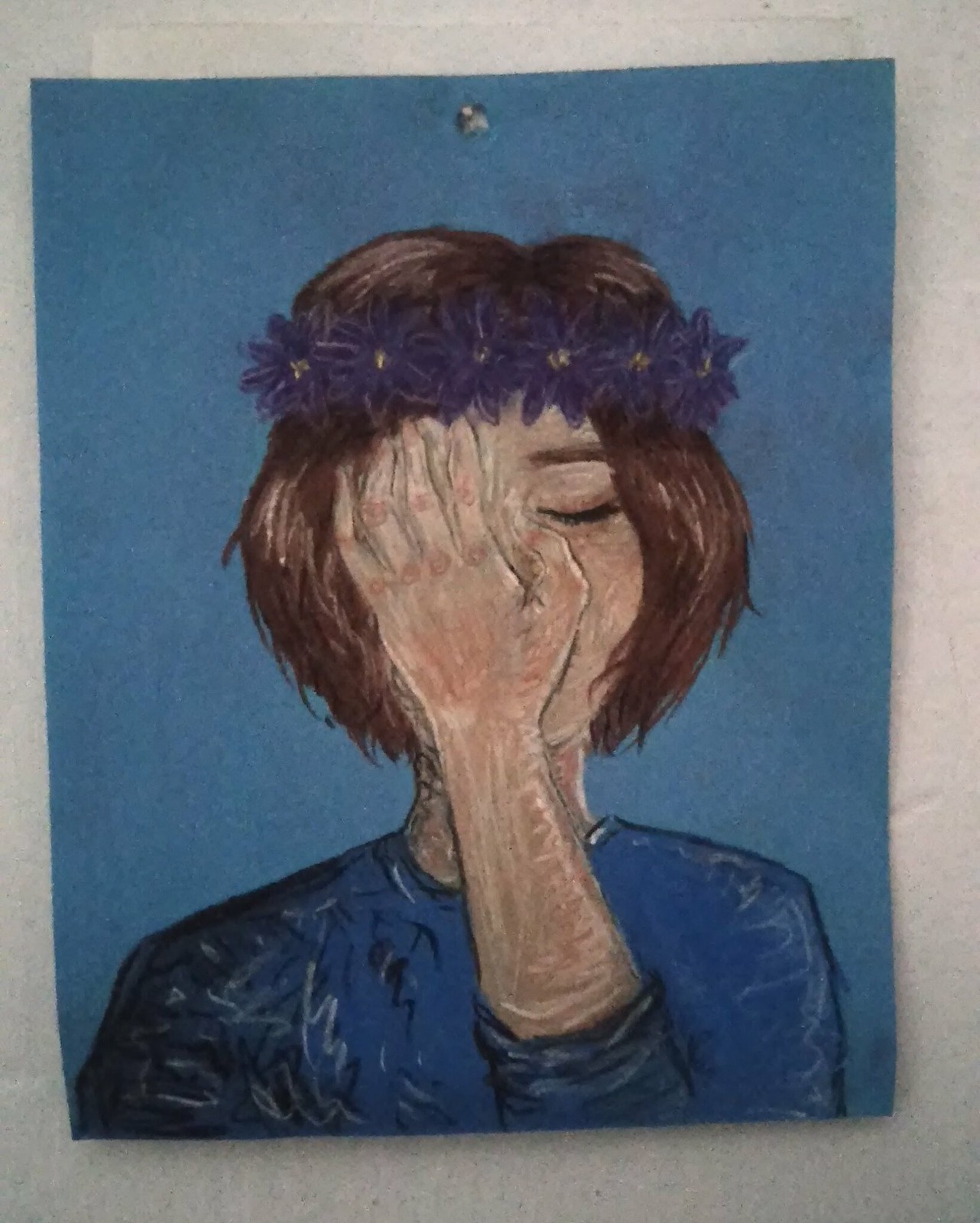This is a detailed photograph of an artwork displayed on a white wall, secured with a gray or clear thumbtack. The image captures a hand-drawn portrayal of a Caucasian woman with a light complexion featuring a mix of peach, pink, and white tones. She has short, chin-length brown hair and is adorned with a floral crown made of purple flowers with gold centers. The woman's right hand covers the left side of her peacefully closed eyes, touching her forehead and partially obscuring her face. Notable pink areas around her knuckles and the base of her fingers suggest delicate skin folding and wrinkling. She is dressed in a dark blue shirt with slightly pushed-up sleeves, showcasing artistic wrinkling effects, rendered possibly using colored pencils or pastels. The artwork's background is a solid dark blue or cyan, contrasting with the white backdrop of the wall where it is displayed. The photograph is taken at a slight angle, revealing the paper to be somewhat diagonal rather than perfectly aligned on the wall. The meticulously detailed depiction includes brown eyebrows and black eyelashes, adding to the character's vivid portrayal.